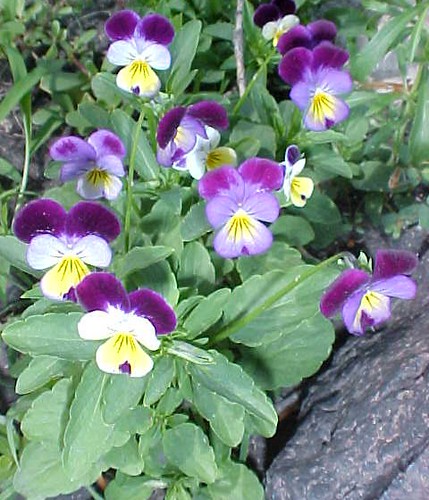In this outdoor, daytime photograph, the focus is on a vibrant garden scene filled with various natural elements. The bottom right corner features a noticeable black rock taking up a triangular portion of the frame. To the left of the rock, several leafy green plants and bushes are visible, providing a lush backdrop. Central to the image are multiple budding flowers with distinct colors of purple, white, and yellow. Notably, a striking flower with two purple petals and three white petals adorned with little yellow sprigs stands out. Scattered throughout the image are about ten other similar flowers, positioned predominantly in the center, with clusters to the left and right as well. The ground beneath the plants is also partially visible, adding to the garden-like setting. The entire image is devoid of text, letters, or numbers, and is captured with high clarity, illustrating the bright and clear natural light typical of midday.